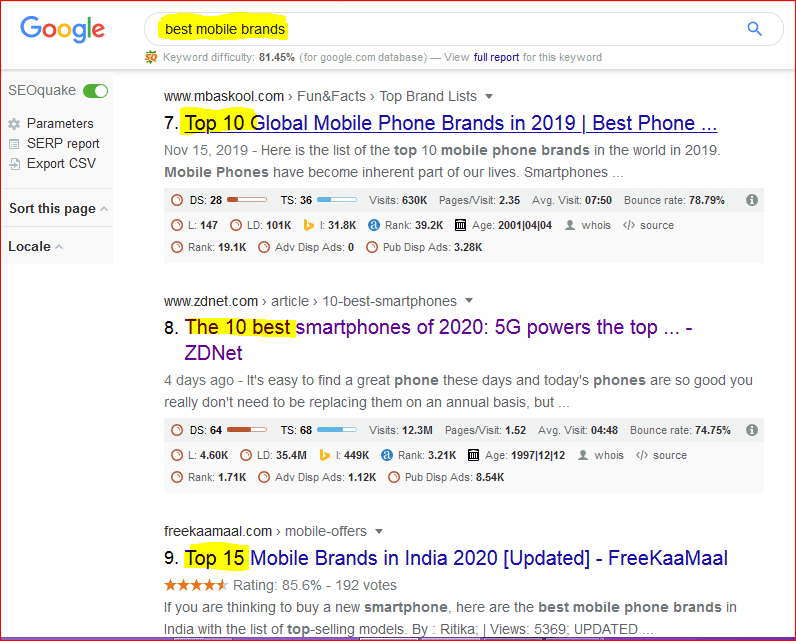This image is a detailed screenshot in landscape mode, surrounded by a prominent red border added by the person who captured it. In the upper left corner, the Google logo is visible, indicating that the screenshot was taken from a Google search results page. 

In the Google search bar, the query "best mobile brands" has been entered and highlighted with a yellow marker for emphasis. Below the search bar, a row displays "keyword difficulty: 81.45%" with an option "view full report" in blue.

On the left side of the screenshot, a sidebar labeled "SEOquake" is present, featuring a green toggle bar. Below it, options like "Parameters," "SERP report," "Export CSV," and "Sort this page" are listed.

In the main section of the screenshot, the search results reveal a list of webpages:

1. The seventh result is titled "Top 10 global mobile phone brands in 2019," highlighted in yellow and displayed in blue text.
2. The eighth result is "The 10 best smartphones of 2020," where "the 10 best" is highlighted in yellow. The snippet below this result mentions "5G powers the top" and is displayed in purple, indicating that it has been visited before.
3. The ninth result is "Top 15 mobile brands in India 2020 updated," with "top 15" highlighted in yellow and the title in blue.

This carefully highlighted and annotated screenshot serves as a visual guide to the search query "best mobile brands," capturing the user’s interaction and areas of focus within the search results.